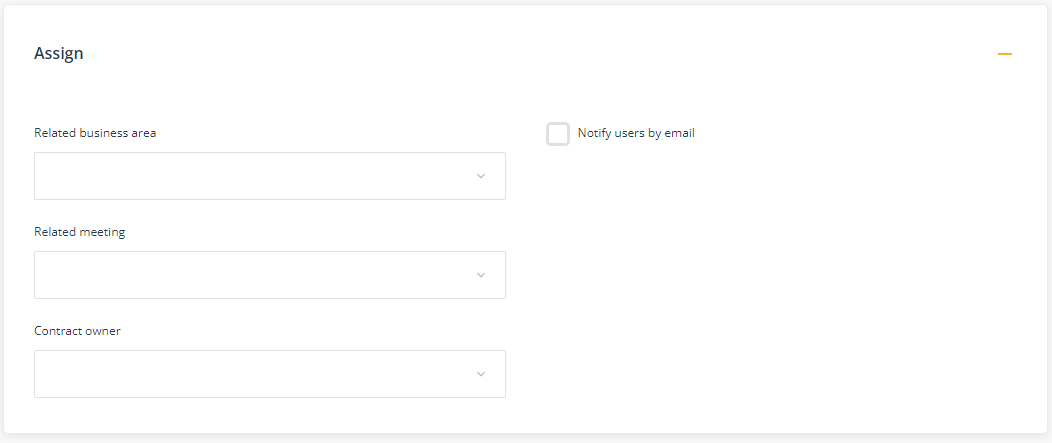The screenshot captures a section of a website interface set against a stark white background, framed by a subtle light gray border. In the upper left corner, the word "ASSIGN" appears in bold, capital letters but smaller print. Directly below, a label reads "Related Business Area," with only the "R" in uppercase, followed by a rectangular drop-down menu indicated by a downward-pointing arrow. Subsequent to this are labels for "Related Meeting" and "Contract Owner," each accompanied by respective drop-down menus.

Centered vertically and positioned towards the middle of the image, aligned with the "Related Business Area" label, there's a light gray-bordered square with a white center. Adjacent to this square is the phrase "Notify Users by Email," with the "N" capitalized, denoting a possible checkbox or clickable field. On the top right segment, just slightly below the top boundary, there's a thin, straight, orange-yellow line running horizontally across. This comprehensive depiction offers a clear understanding of the features and layout of the website interface.